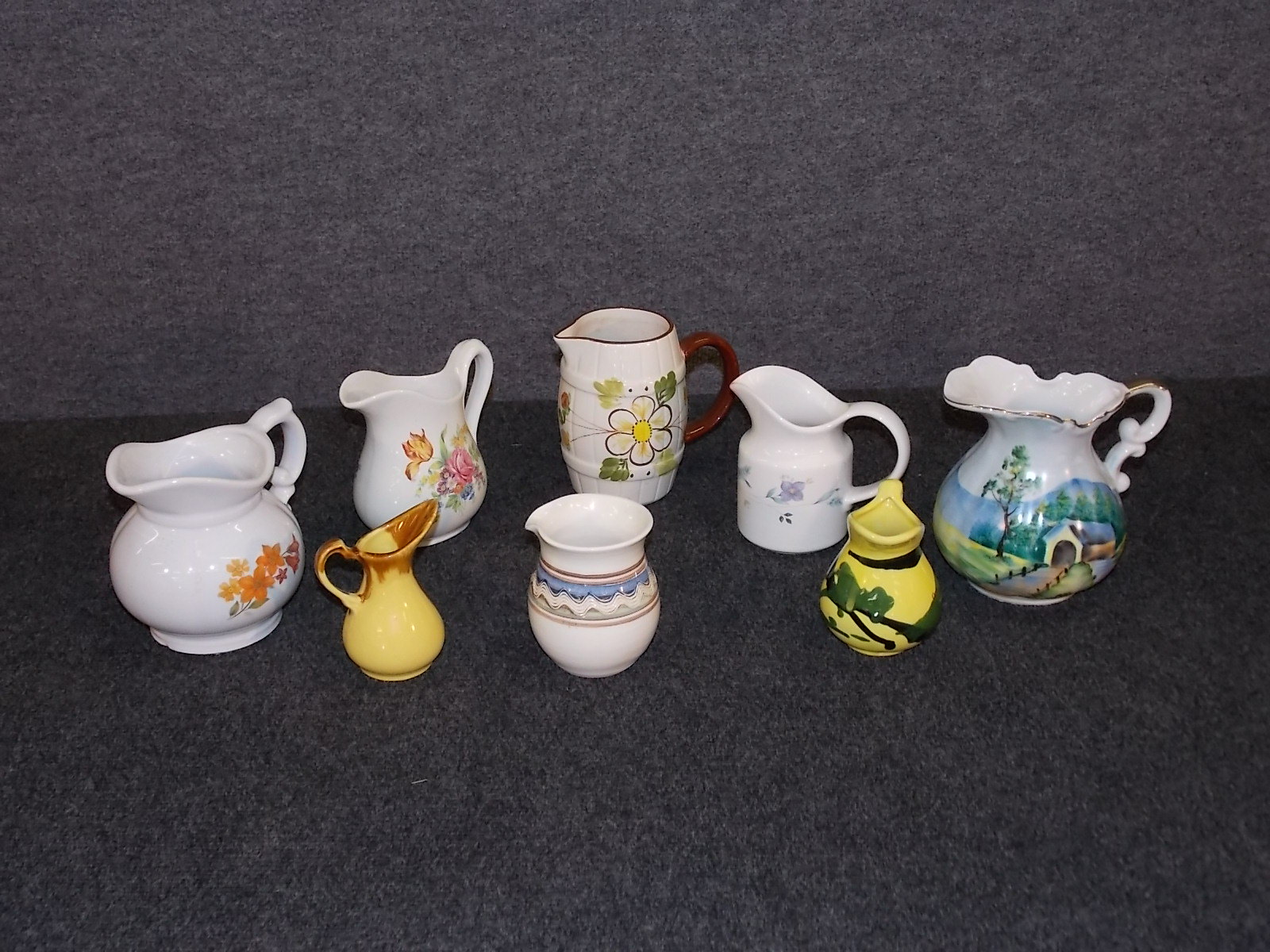The image is a detailed indoor photograph featuring a small collection of eight decorative ceramic pitchers, arranged on a plain dark grey fabric background that matches the wall behind them. Most of these pitchers are white, with six exhibiting varying floral patterns in shades of orange and pink, and one having a simple wave design. The other two pitchers stand out with their bright yellow color; one adorned with brown accents, and the other with greenish-black patterns. Among the white pitchers, one uniquely features an intricate painted scene of a house with a tree, while another showcases a landscape with a covered bridge and mountains. Most pitchers have handles, with one particularly ornate. Their shapes vary from wide-bodied to more column-like structures, but they all serve the purpose of pouring various liquids.